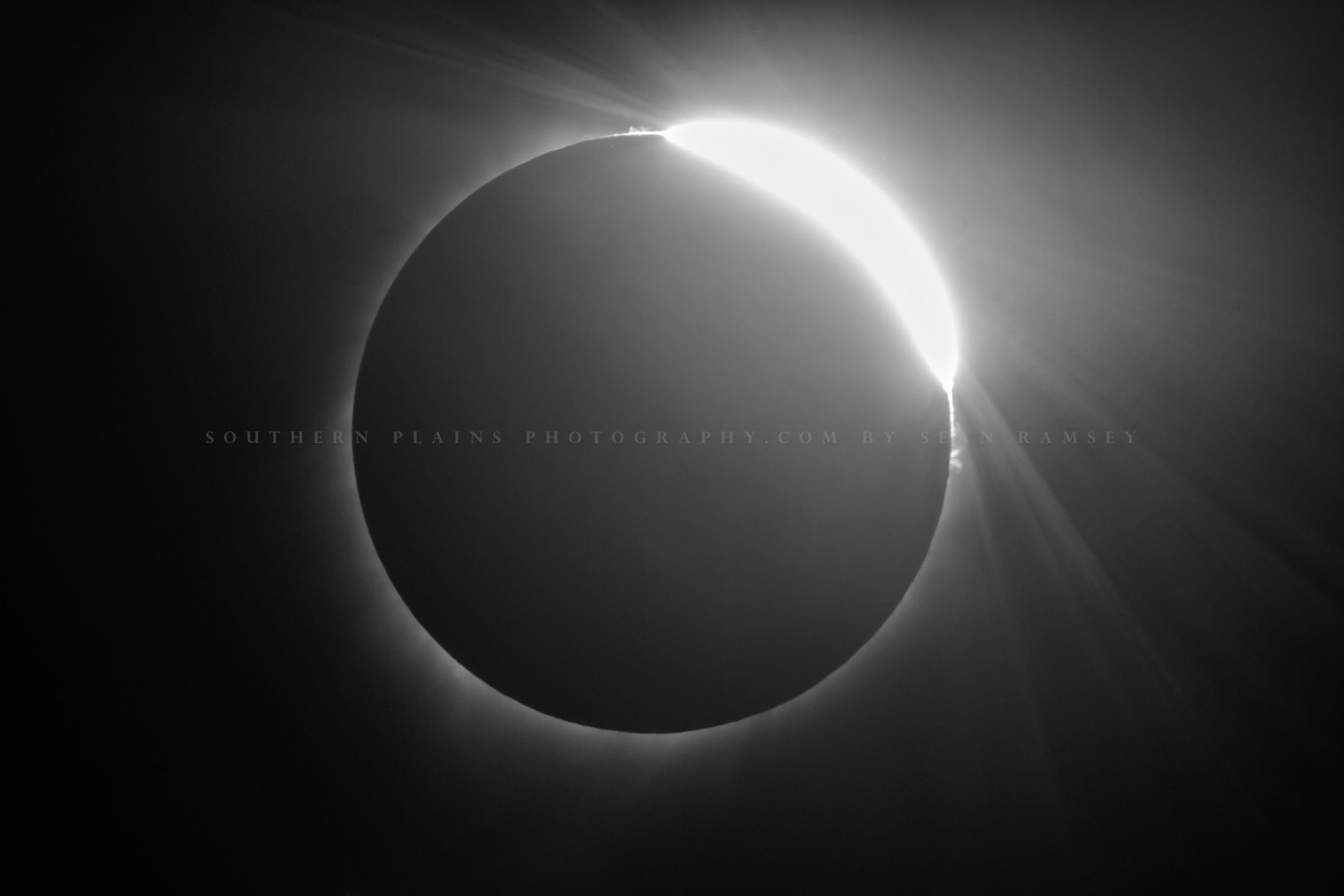This black and white photograph captures a partial solar eclipse. The moon predominantly obscures the sun, leaving a crescent of sunlight visible in the upper right quadrant. Stark contrasts define the image, with the black background sharply highlighting the sun's bright light. Rays from the exposed part of the sun emanate towards the edges of the rectangular image, creating an intense visual effect. A faint gray watermark reading "southernplanesphotography.com by Sean Ramsey" stretches across the center, although part of the name 'Sean' is slightly obscured by light rays. Overall, the eclipse is centered both horizontally and vertically, allowing ample space around the main event and emphasizing the dramatic interplay of light and shadow.